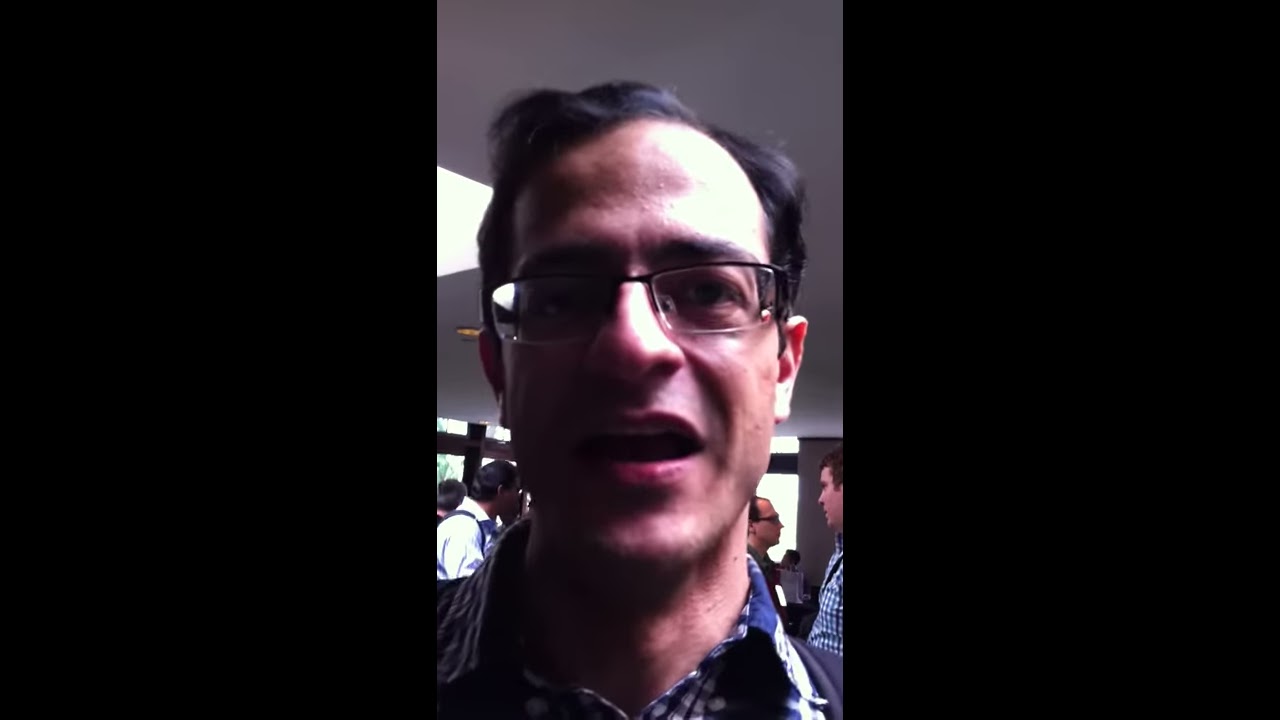The focal point of this image is a man directly in the center, staring into the camera. He has somewhat pale skin, dark wispy hair parted to the right, and thick, black eyebrows. He wears black-framed eyeglasses that sit on a long, angular nose. His ears are small and slightly pointy. He has a partially open mouth showing his upper teeth but no visible lower teeth. The man has a long neck and wears a blue plaid button-down shirt with a collar, possibly patterned, suggesting he may also be carrying a backpack. The scene is set indoors, likely during the day, possibly in an office or convention setting, as suggested by the white ceiling with overhead lighting and windows visible in the background. Surrounding the main subject, towards the bottom and background of the image, are three other men engaged in conversation. These men, all Caucasian, add context to the scene, underlining its conversational and perhaps professional nature. The image is framed with black on both the right and the left sides.